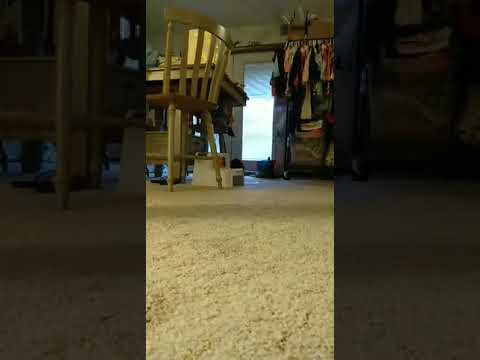This image portrays an indoor setting, likely captured from a low angle, possibly from a security camera or a floor-level perspective in a living room or dining area. The scene is dominated by a short, tan plush carpet that spans the floor, and the space is relatively sparse with a few distinct objects and furniture pieces.

Prominently located towards the top center of the image is a large, white, double French door with glass window panes that seem to overlook a backyard. The window blinds are partially pulled down. In front of these doors, there is a light wooden chair positioned to the left, adjacent to a wooden table which holds various objects. To the right of the chair sits a white step stool.

On the right side of the image, near the doors, stands a tall, wooden coat rack with multiple jackets and pieces of cloth draped over it, featuring a mix of colors including red, light blue, and black. Below the coat rack, there is a clear storage bin filled with more clothing items, contributing to a makeshift storage area. Overhead, a ceiling lamp or fan with a light fixture can be seen.

The overall scene is set indoors, characterized by a blend of neutral colors like tan, light brown, and white, with pops of color from the hanging garments. The perspective suggests a domestic and cozy environment focused around the entryway to the house.